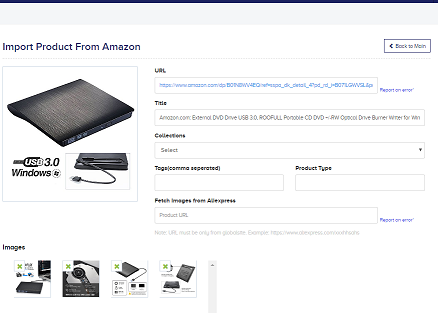This image displays an order page interface for importing products from Amazon. Occupying the top section of the page, on a clean white background, there is a header that reads, "Import Product from Amazon." Just beneath this, there's a primary image showcasing what appears to be computer equipment. Initially, it seems to resemble a large square device, possibly a router or a networking apparatus, but further inspection reveals it is actually an external DVD drive, labeled "USB 3.0 Windows."

At the bottom section, additional images provide various angles of the same external DVD drive to offer a comprehensive view of the product. Adjacent to the primary image at the top, on the right side, there is a text box labeled "URL" where users can input the URL of the desired Amazon item. Below this, the field labeled "Title" further clarifies the product as an external DVD drive.

Further down, there is a dropdown menu under the "Collections" option, allowing the user to categorize the product within specific collections. The next section is labeled "Tags," followed by a box for specifying the product type. Near the bottom of the interface, there is a heading titled "Fetch Images from AliExpress," accompanied by another text box designated for inputting the product URL to retrieve images from AliExpress. This detailed layout aims to streamline the process of importing and categorizing products efficiently.